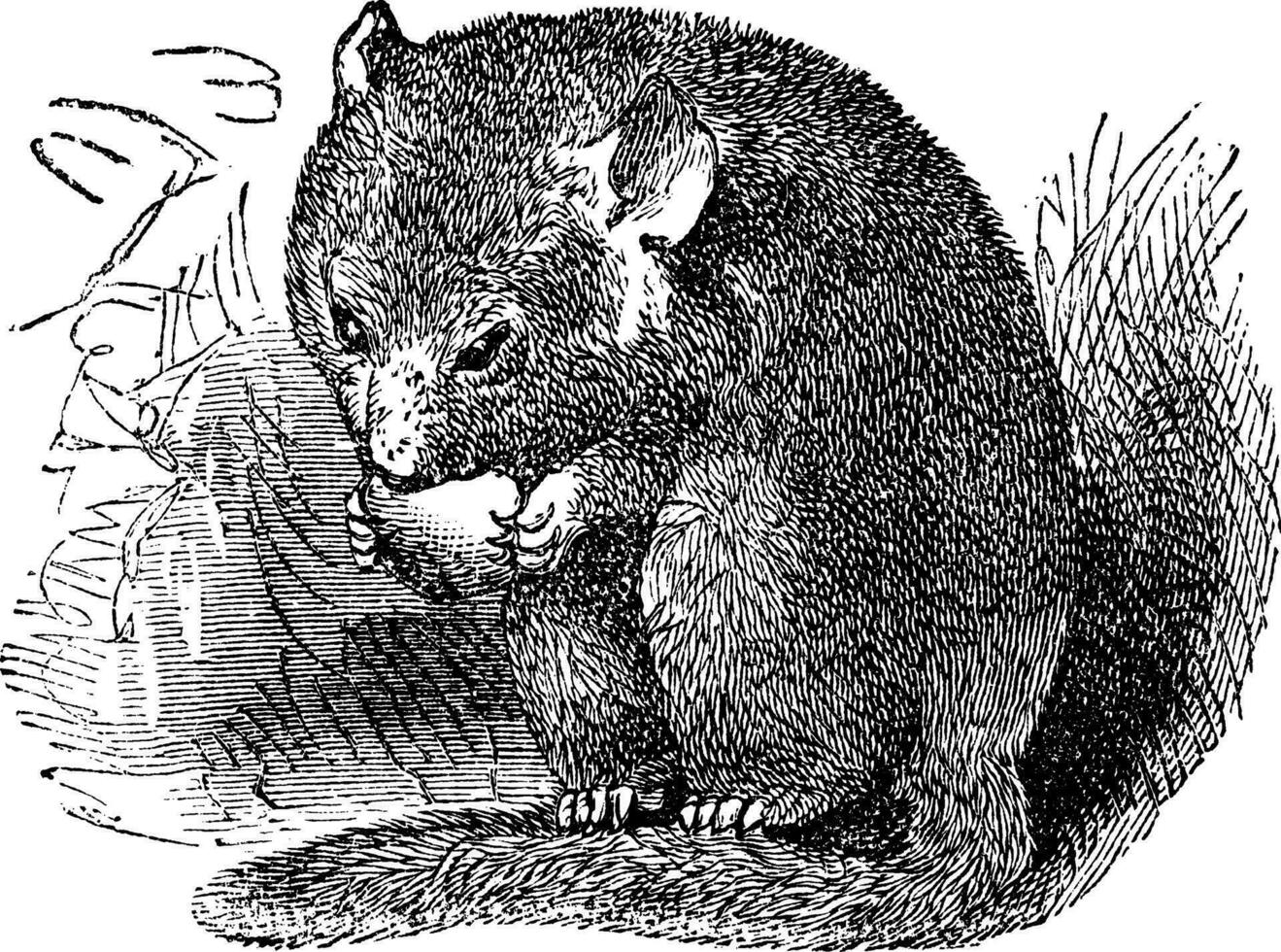This is a detailed digital line drawing in black and white, featuring a beaver that is hunched over while eating a piece of fruit, which it holds between its front paws. The beaver is in a sitting position, with its flat tail wrapped around its feet. The background is composed of simple lines and shaded patterns, emphasizing the monochromatic theme. The beaver is the central focus of the drawing, outlined with precise black lines against the white backdrop. Despite the minimalistic setting, the detailed inked shading vividly depicts the texture and form of the beaver and its surroundings.